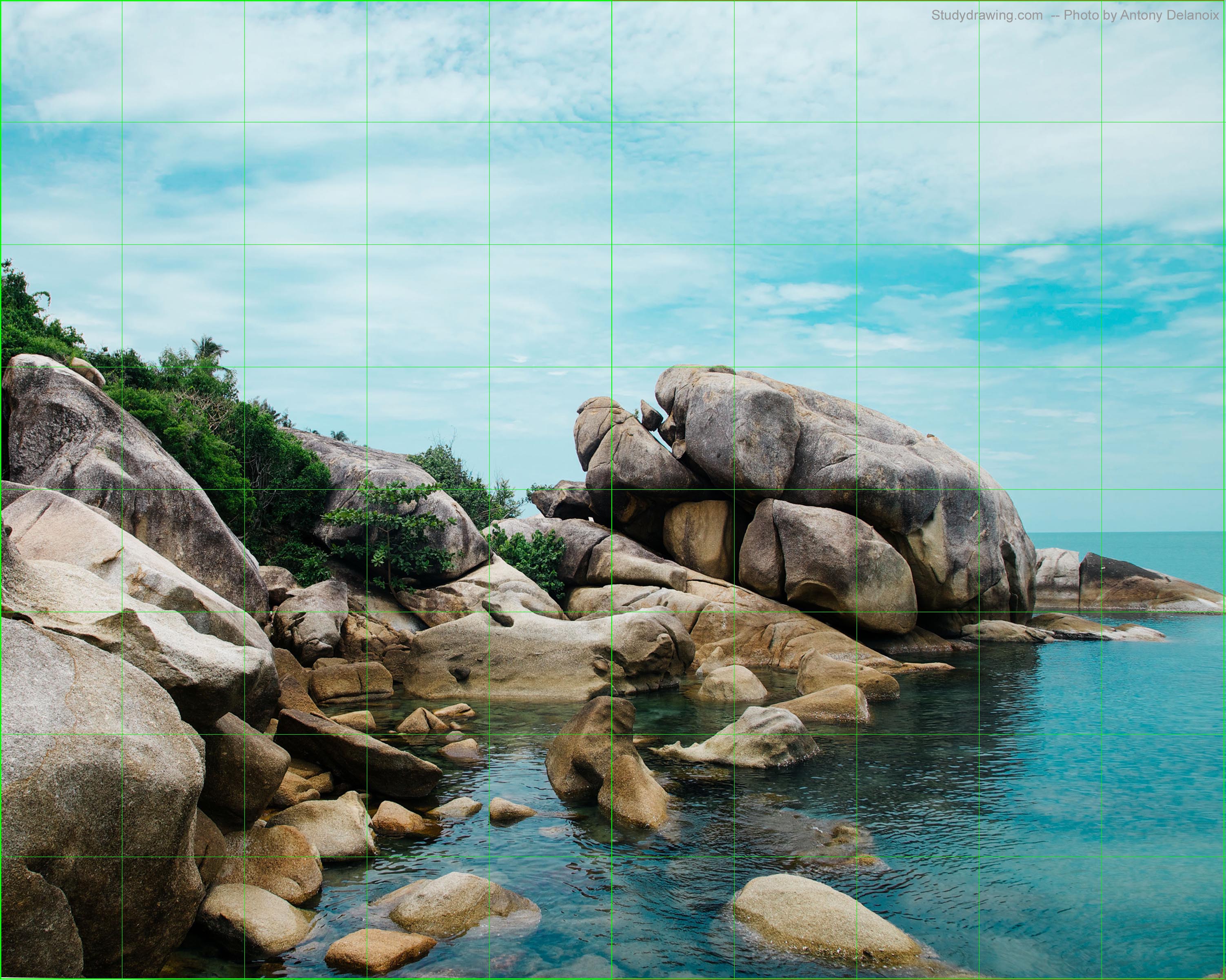This is a detailed color photograph of a rocky seacoast, featuring a rugged outdoor setting divided by subtle, green rectangular grids that aid in drawing. The scene showcases large gray and brown boulders on the left, interspersed with green herbs and plants forming a sloping terrain. The water, with its blue and greenish-blue tint, surrounds the rocks, some of which are submerged. Toward the right, a prominent large rock is surrounded by slightly smaller rocks, extending into the sea. The backdrop is a blue sky adorned with white and gray clouds. In the top right corner, small grey text, possibly reading "studydrawing.com," credits the artist behind the photograph. The image, resembling a stylized landscape, might function as a jigsaw puzzle with an intricate and vibrant coastal theme.